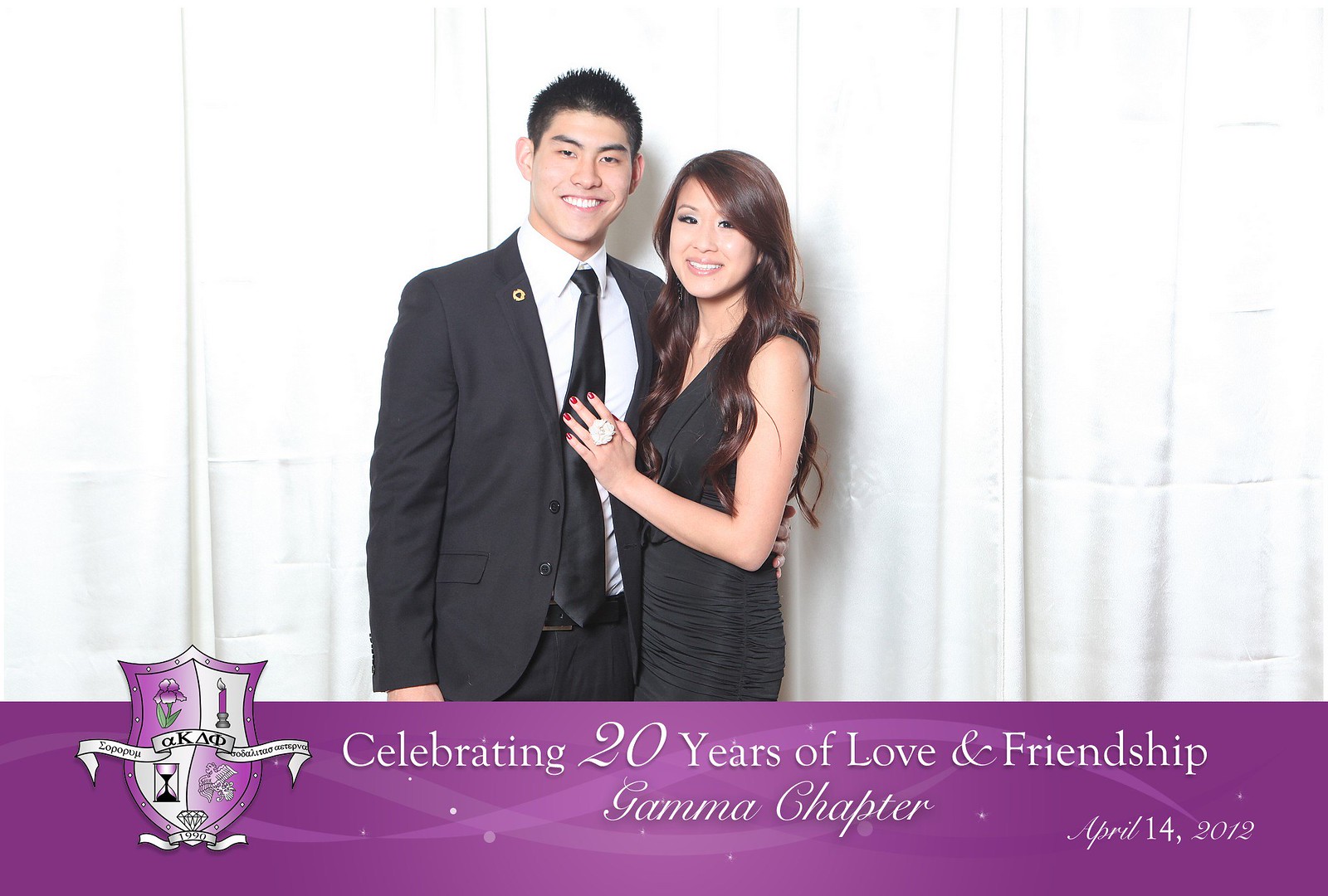This color photograph depicts an Asian couple dressed in coordinated semi-formal black attire, standing against a white backdrop curtain. The man, positioned on the left, wears a black suit with a black tie and a white dress shirt, accessorized with a gold lapel pin. The woman, standing on the right, is adorned in a black dress, sporting long dark brown hair and red nail polish. She has a prominent diamond ring on the middle finger of her left hand, which she rests on the man's chest. They both smile warmly at the camera, exuding a sense of joy and connection.

Below the image, a purple banner spans the entire width, marked on the left by a crest and on the right with white text. The crest is divided into four quadrants, each depicting icons—likely a purple flower, a purple candle, an hourglass, and a purple mythical creature. The text beside the crest reads, "Celebrating 20 Years of Love and Friendship, Gamma Chapter," with the date "April 14, 2012" displayed in a mix of cursive and italicized fonts.